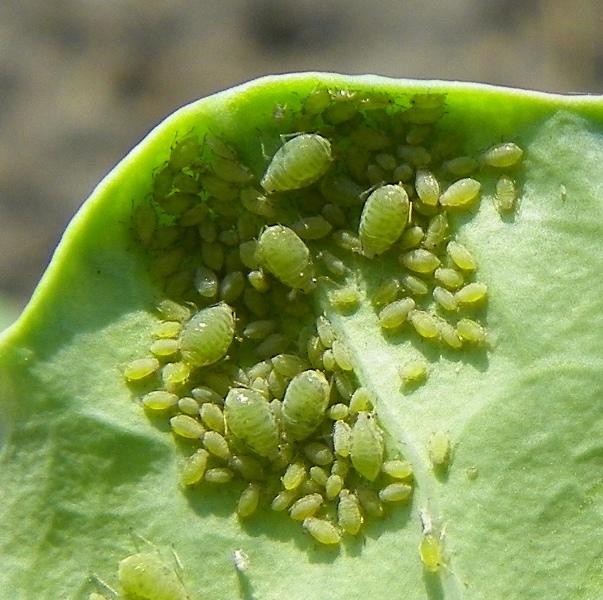The image is a vibrant close-up, likely a macro photograph, of a lush green leaf that dominates almost the entire frame. The leaf extends from the middle left, swooping upward to the right and then flattening out horizontally, stretching off the image at various points including the lower left and bottom. The background is blurry and dark, hinting at an outdoor setting with strong daylight. The leaf is a vivid lime green, teeming with numerous small, oval-shaped larval insects, possibly larvae, concentrated primarily in the upper middle and descending to the left. Scattered among these are several larger green bugs with segmented bodies featuring horizontal light green lines. The image is densely populated with these insects, creating a scene of active inhabitation and possibly egg-laying.